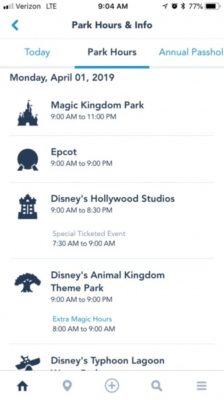The screenshot depicts an information screen on a smartphone, featuring various details. At the top, the phone shows a connection status of 2 out of 4 bars with Verizon LTE, the time as 9:04 AM, and a battery level of 77%. An arrow pointing left is also visible. The highlighted section contains "Park Hours and Info" with today’s date specified. The date displayed is Monday, April 1st, 2019. Beneath this, the screen lists different Disney theme parks along with their operating hours:

1. **Magic Kingdom Park**: Open from 9:00 AM to 11:00 PM, accompanied by an image of a castle.
2. **EPCOT**: Open from 9:00 AM to 9:00 PM.
3. **Disney's Hollywood Studios**: Open from 9:00 AM to 8:30 PM, with a special ticketed event from 7:30 AM to 9:00 AM.
4. **Disney's Animal Kingdom Theme Park**: Open from 9:00 AM to 9:00 PM, with Extra Magic Hours from 8:00 AM to 9:00 AM.
5. **Disney's Typhoon Lagoon**: Name listed with an icon next to each park.

Each park listed has an associated icon on the left side for easy identification. The highlighted, bolded, and underlined text "Part Hours" in blue indicates the selected section on the information screen.